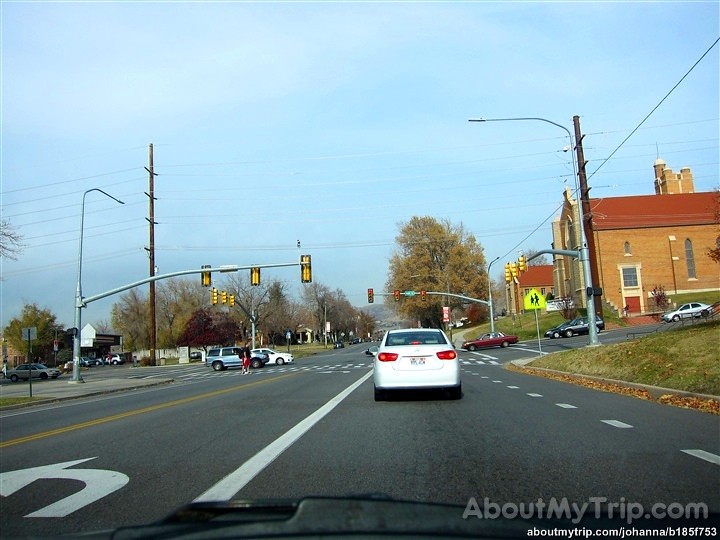This is a brightly lit, daytime photograph taken from inside a car, looking out through the windshield at a bustling intersection. In the foreground, part of the vehicle's dashboard is visible at the bottom of the frame. The scene ahead features a two-lane road with a left turn lane adjacent to the vehicle and a single lane for oncoming traffic. Directly in front, a white car is stopped at the intersection.

Numerous cars can be seen in motion as they navigate the crossing ahead, along with a pedestrian making their way through the crosswalk. The road extends straight into the distance under a clear, blue sky. On the corners, there are brick buildings, and multiple trees line both sides of the road, adding a touch of greenery to the urban landscape.